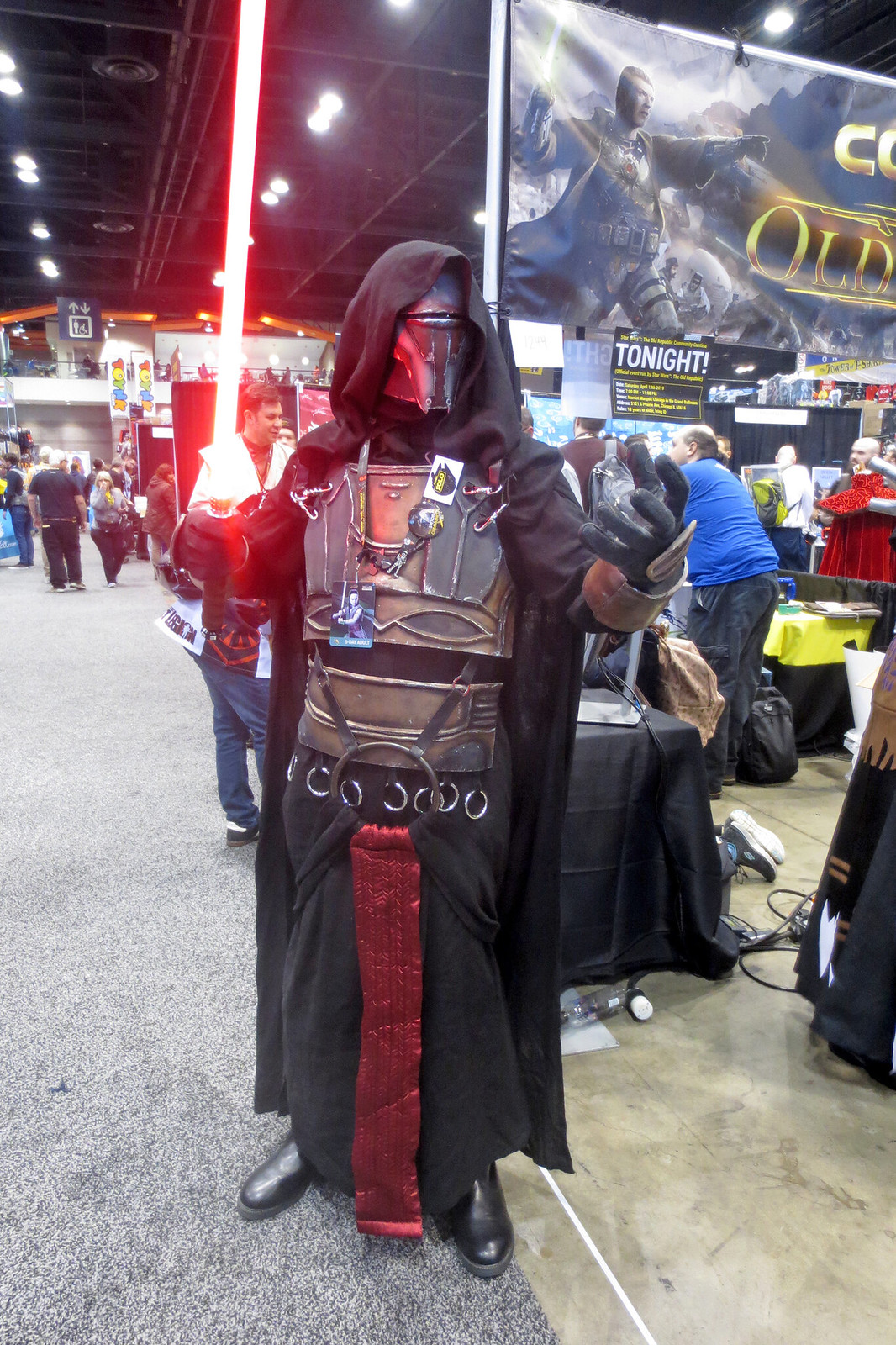In the bustling hub of a convention center, surrounded by tables, crowds, and stands, stands an imposing figure in elaborate cosplay. The character, reminiscent of Darth Revan from the Star Wars universe, is clad in dark black robes with intricate bronze and metallic armor patterns. A striking red banner hangs down the front, positioned between his legs. His chest and torso are guarded by armor, and he dons a silver mask and metallic helmet with a thin black horizontal visor, all beneath a black hood.

This captivating figure is captured mid-pose, with his right hand extended forward in a dramatic grabbing motion, as if summoning the Force, while his left hand confidently grips a bright red lightsaber, held just above his chest and to the side. He gazes to the right, as if lost in character.

Behind him, the convention center is alive with activity, featuring a large poster in the top right corner that showcases a similar character wielding a lightsaber and extending an arm, echoing the cosplayer's stance. The ceiling lights and visible corridor add depth to the scene, highlighting the vibrant atmosphere of this immersive Star Wars-themed spectacle.